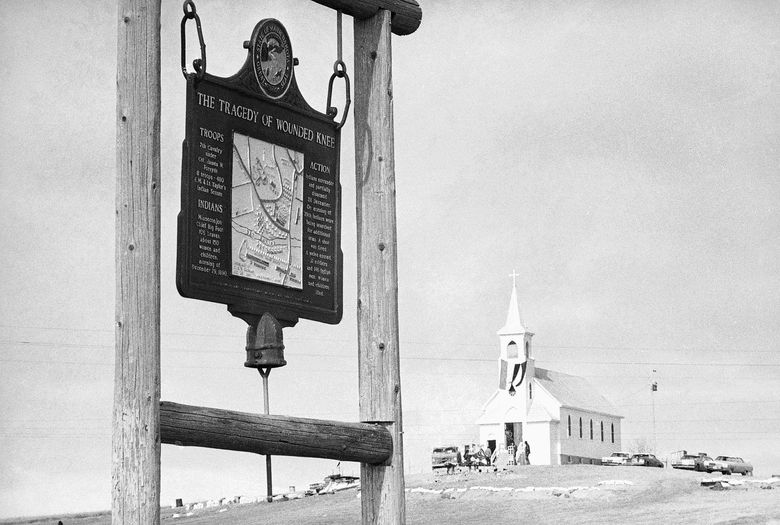The black-and-white photograph, in a landscape layout, intricately captures a poignant scene of historical reflection. Dominating the foreground is a large wooden frame supporting an informational placard entitled "The Tragedy of Wounded Knee." This placard, featuring a central map, is divided into three distinct sections labeled "Troops," "Indians," and "Action," although some text is illegible. The detailed map and categorized information aim to teach viewers about a significant event in history.

In the background, perched atop a dirt hill, stands a small, white church adorned with a steeple topped by a cross. This church, with its five windows on each side, appears serene yet stark amidst the somber context of the placard. Surrounding the church are several parked cars, and a group of people is gathered on the steps leading up to its entrance, adding a human element to the scene. The day seems overcast, as indicated by the thick cloud cover in the sky. Additionally, wires and poles are visible, hinting at a sparse yet connected community. The photograph, with its layers of detail and juxtaposition of historical narrative against a peaceful setting, invites deep reflection on the events that took place at Wounded Knee.